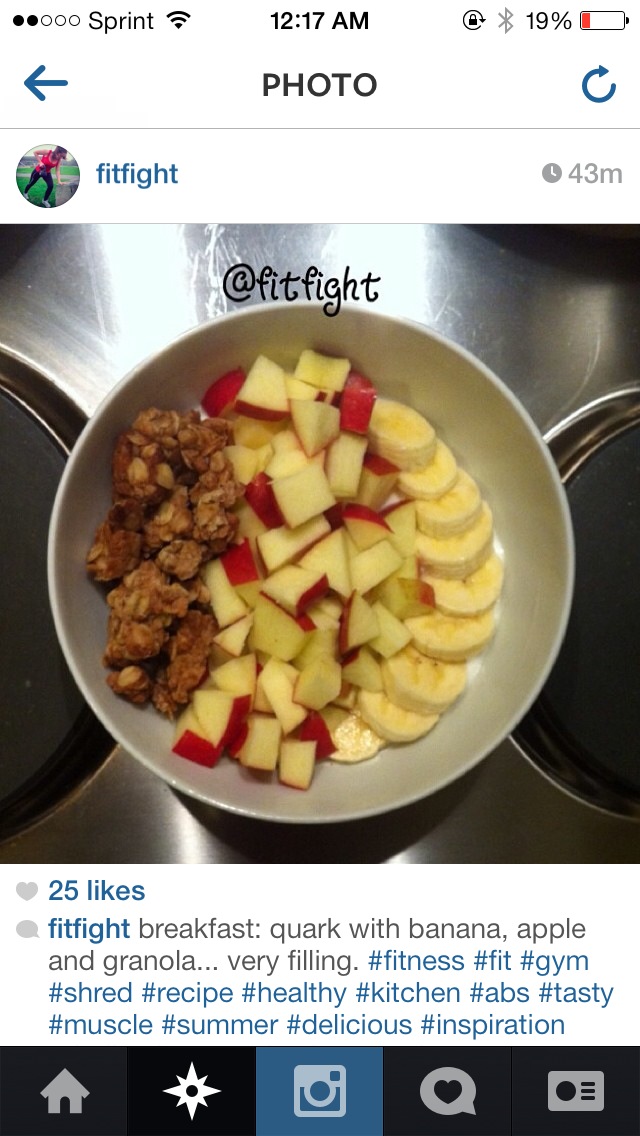This Instagram post by user Fit Fight features an overhead photograph of a nutritious breakfast bowl filled with sliced bananas, cubed apples, and crunchy granola, all set against a metallic surface. The profile of Fit Fight, identified by a small circular icon of a woman in red, is displayed at the top. The header shows it is 12:17 a.m., with a battery level of 19% and connected to Sprint’s Wi-Fi. The post, uploaded 43 minutes prior, has garnered 25 likes. The caption reads: "Fit Fight breakfast crock with banana, apple, and granola. Very filling." It is followed by several hashtags emphasizing health and fitness, including #FitFight, #Fit, #Gym, #Shred, #Recipe, #Healthy, #Kitchen, #Abs, #Tasty, #Muscle, #Summer, #Delicious, and #Inspiration. The Instagram interface is evident with icons for home, navigation, photo, heart, and speaker visible in the footer.